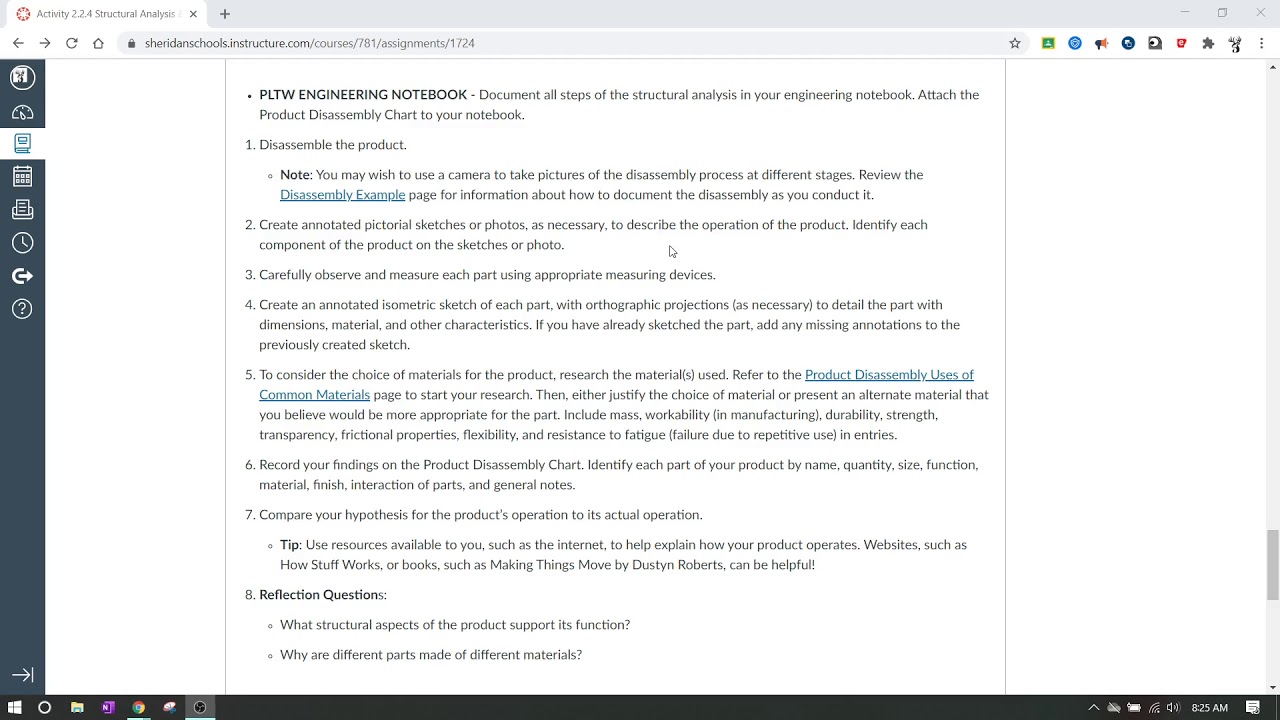The screenshot depicts an educational online activity, seemingly designed for a class focused on structural analysis. It features a user interface with a small logo labeled "Next Activity" in the corner and a predominant white background, upon which a detailed instructional sheet is displayed. The document is titled "PLTW Engineering Notebook" in bold black font.

The instructions on the sheet outline a step-by-step guide for students to document the disassembly and analysis process of a product. It advises students to:

1. Disassemble the product while photographing the process at various stages.
2. Create annotated pictorial sketches or photos to describe the operation of the product, making sure to identify each component.
3. Carefully observe and measure each part with appropriate measuring devices.
4. Produce annotated isometric sketches of each part along with orthographic projections.

The document's objective appears to be to help students comprehensively document and understand the structural components and functionality of a product. This exercise is part of their engineering studies aimed at developing critical analytical and documentation skills. The activity concludes with a reflection question, encouraging students to synthesize and evaluate their findings.